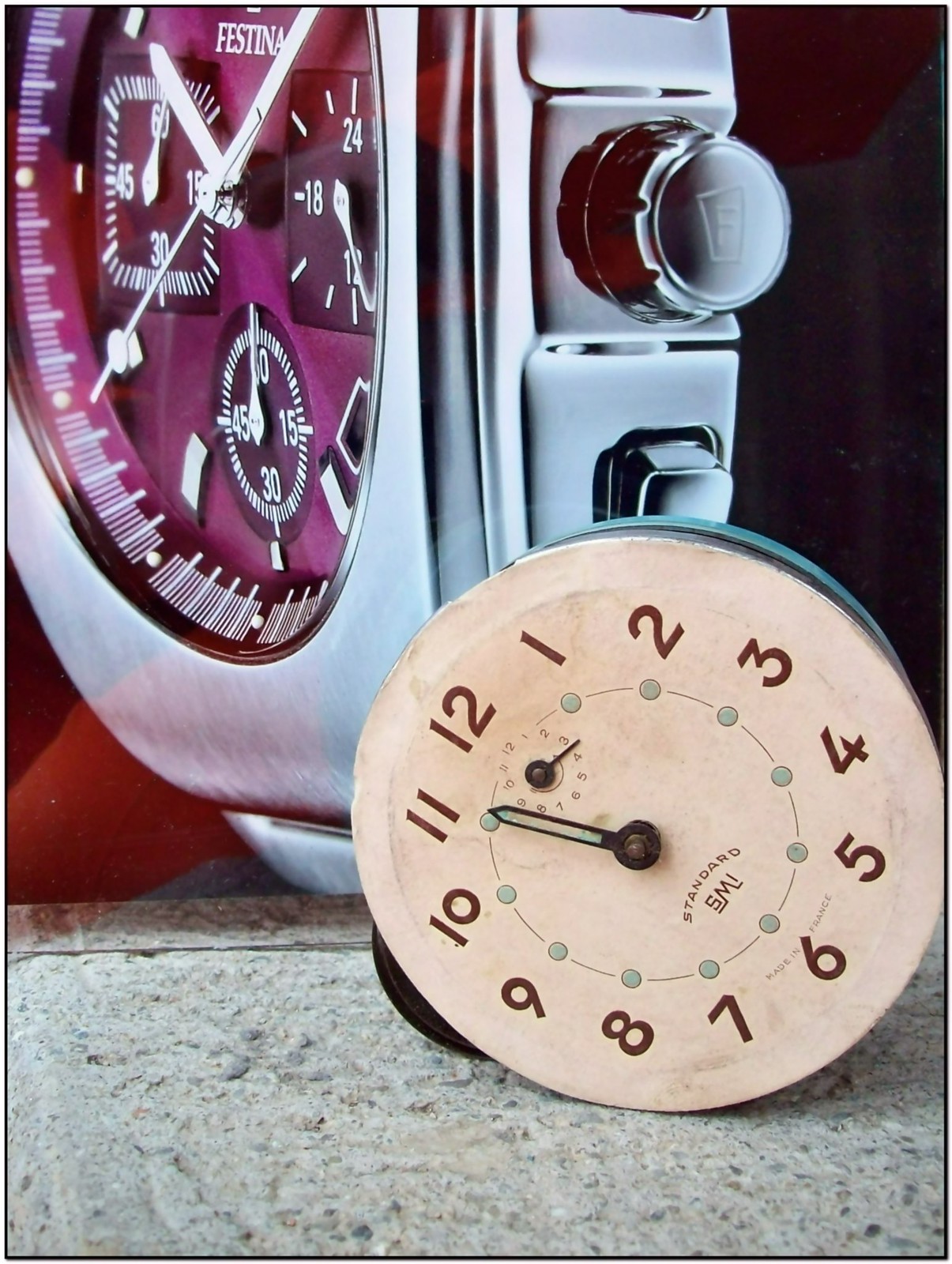A photograph captures a juxtaposition of timepieces, each with its own unique charm. In the foreground, an aged clock proudly displays its yellowed, paper-like face, adding a vintage touch to the scene. The clock, marked by the brand "Standard SMI," features burgundy or brown numerals from 1 to 12, though it only retains a single minute hand, hinting at the passage of time and wear. Behind this vintage clock, a large and striking display poster showcases a modern wristwatch. This wristwatch, a model by the brand Festina, boasts a sleek brushed stainless steel exterior paired with a captivating purple face, offering a stark contrast to the old-world charm of the foreground clock.